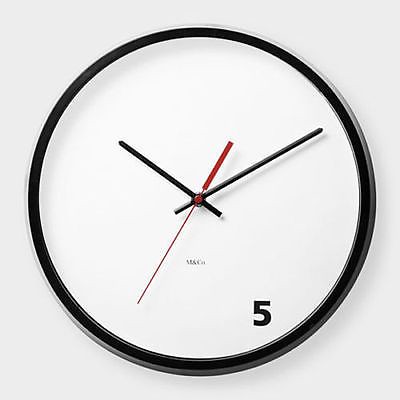This is an image, likely a computer-generated rendering, of a black-framed, round wall clock set against a white square background with subtle gray shadowing. The clock's face is white, featuring only one number, a black "5," while the rest of the dial remains blank. The clock's hands are distinctive: two black lines indicating the hour and minute, and a red line marking the seconds. Below the clock hands, there is some small, unreadable black font. The clock has a slight gray shadowy tint around its edges, reinforcing its three-dimensional appearance. Overall, the scene is minimalistic, with no other objects present, emphasizing the simplicity and abstract nature of the clock design.